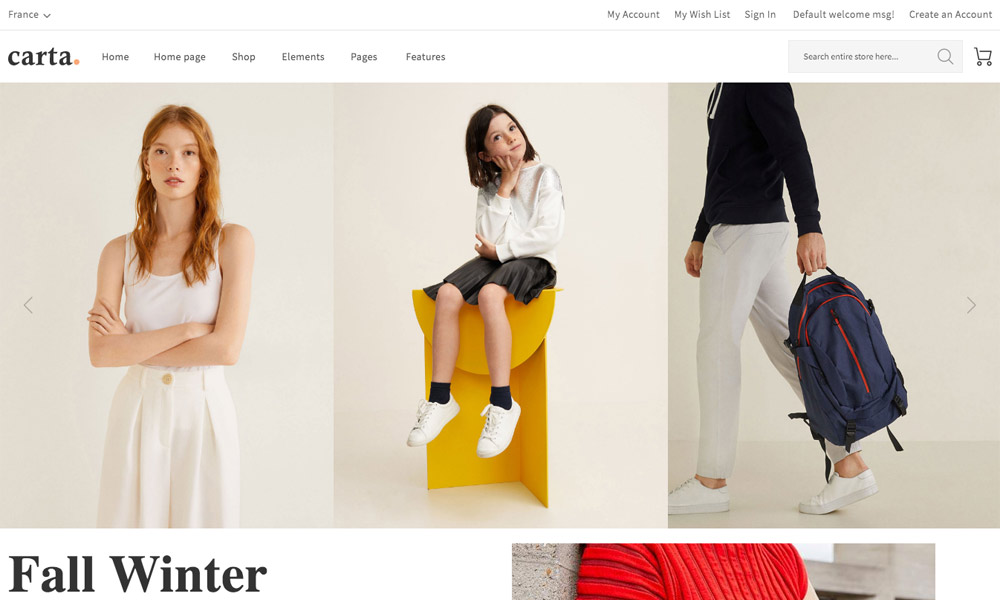The image depicts a website interface that is approximately 1.5 to 2 times wider than it is tall. In the upper left corner, the country selection is set to "France," accompanied by a dropdown arrow indicating the option to change the country. On the upper right, the navigation menus are right-aligned and include options such as "My Account," "My Wishlist," "Sign In," a default welcome message, and "Create Account," separated by a horizontal line from the rest of the content.

The logo, positioned in the upper left, is prominently displayed in bold black font reading "Carta," with an orange diamond symbol situated to the right of the 'A,' roughly a third of the logo's height. Adjacent to the logo is the main navigation menu, rendered in medium gray text, featuring links labeled "Home," "Homepage," "Shop," "Elements," "Pages," and "Features." To the right of this main navigation is a search bar with a shopping cart icon. The search bar has a light gray background with darker gray text prompting users to "Search entire store here..." alongside a gray magnifying glass icon.

Below the header and navigation area, the main section of the site displays three images of models wearing clothing, indicating the website’s focus on fashion.